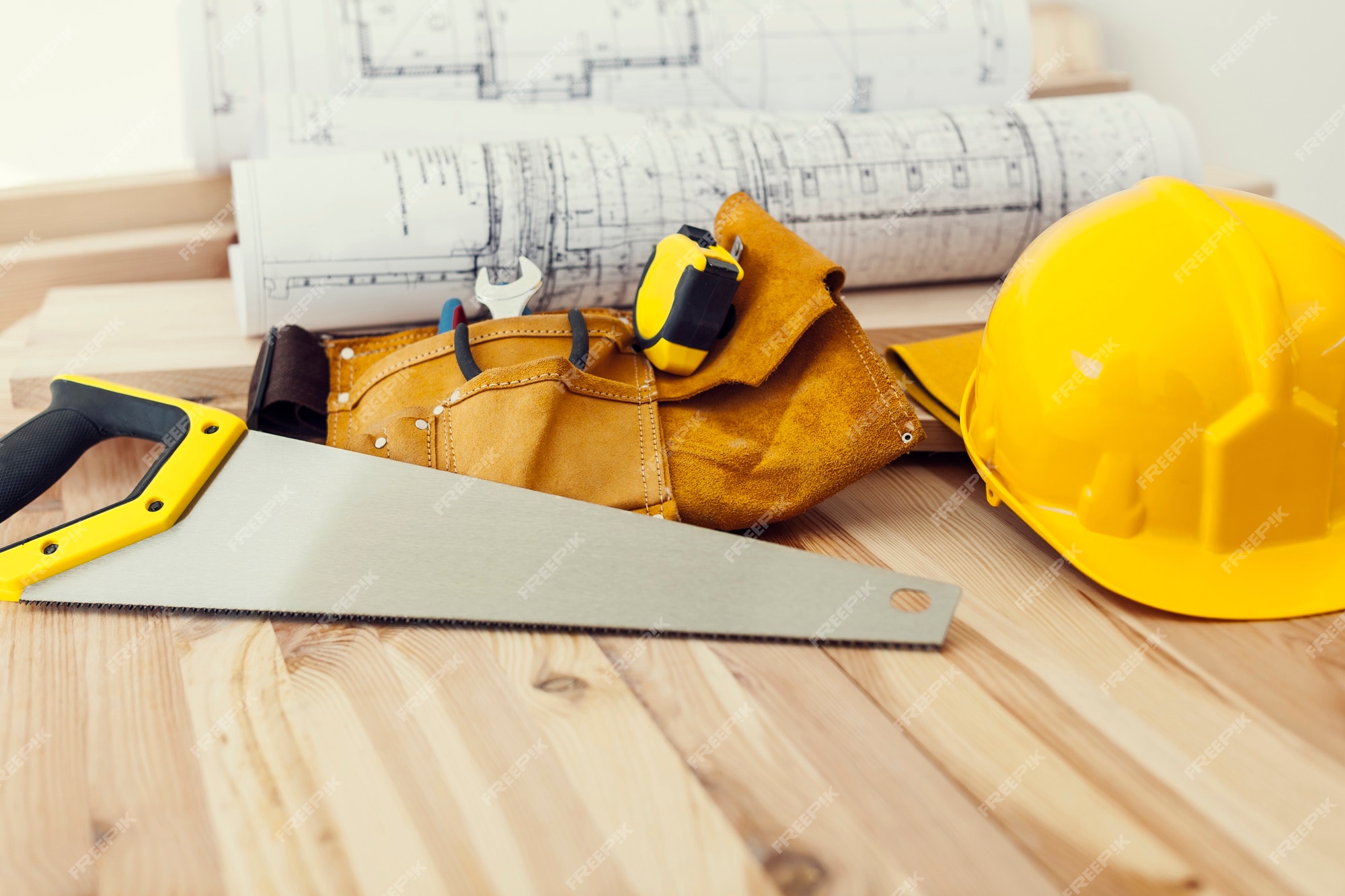This stock image captures an assortment of construction tools neatly arranged on a wooden floor composed of planks oriented towards the top-right. In the foreground, a saw with a yellow and gray textured handle lies prominently. Adjacent to it on the right is a bright yellow hard hat. Centrally positioned is a pristine leather tool belt equipped with various instruments: a wrench, a tape measure, pliers, and what might be a screwdriver. Behind the saw and belt, a couple of rolled-up blueprints with black diagrams sit against a white wall in the backdrop. The overall scene suggests a well-organized workspace ready for construction activities.